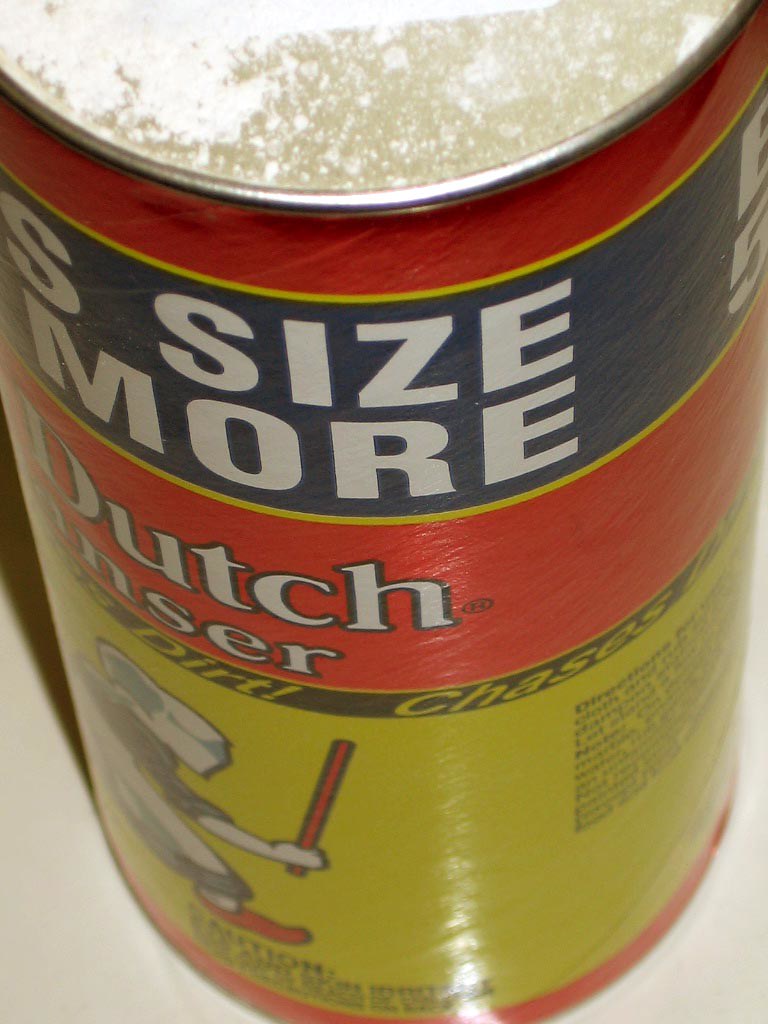This close-up image captures the top portion of an aluminum can, showcasing intricate details. The top of the can is adorned with a fine, powdery white substance. The can itself features a vibrant color scheme with a red and yellow base. Prominently displayed is the image of a man holding a stick, wrapped around by a blue ribbon that partially conveys the letter "S." Alongside, there's white text and visible letters "Dutch N-S-E-R" set against the colorful background. Below this, a black ribbon can be seen with bold yellow text highlighting the word "Dirt!" An exclamation point discreetly seats next to more text, partially obscured and unreadable, adding to the mystery of the imagery.